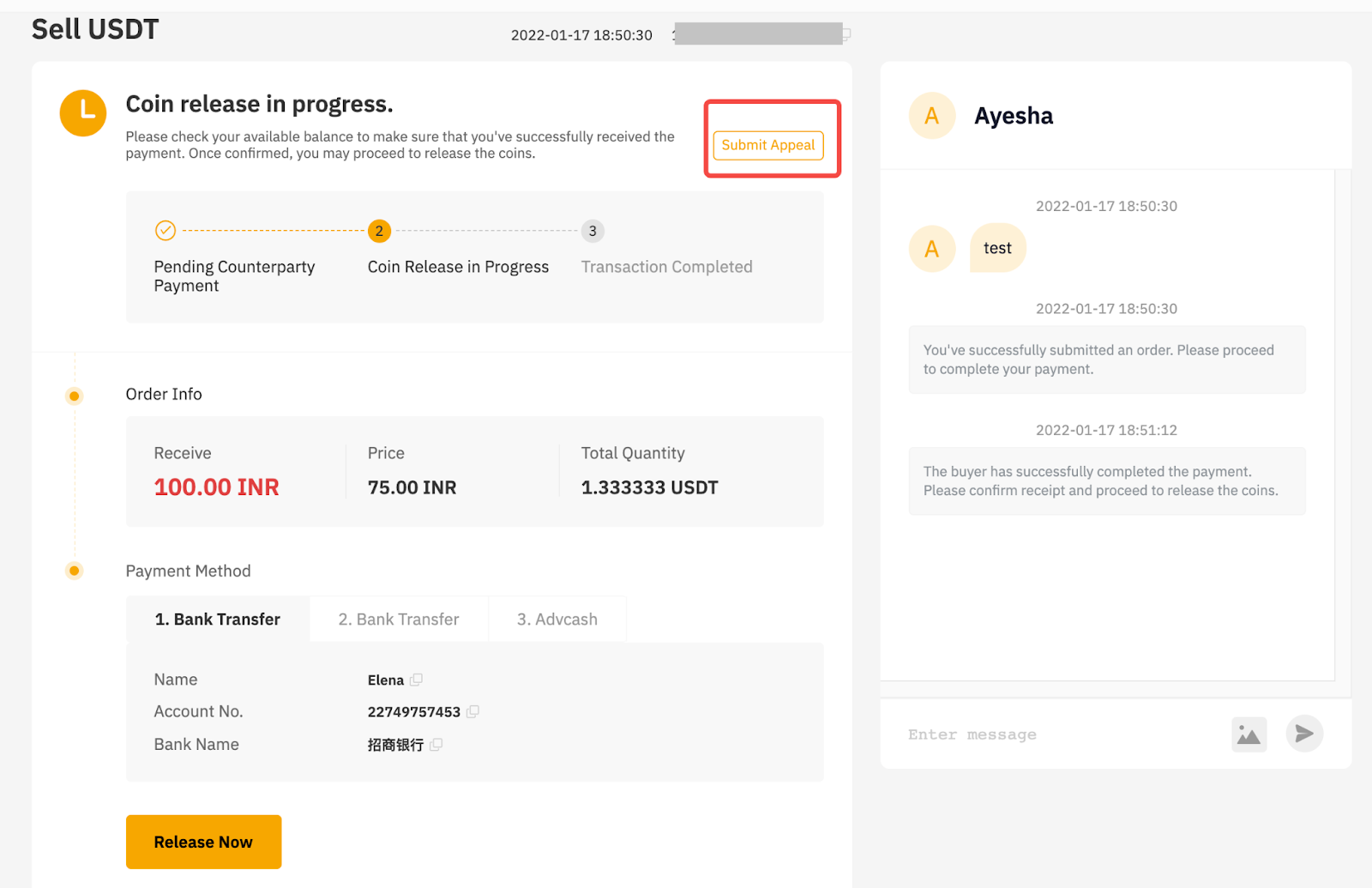The screenshot captures a transaction interface for selling USDT on a cryptocurrency platform. 

In the top left corner, the title "Sell USDT" is visible. The top section of the screen displays the date, an image of a clock, and the message, "Coin release in progress. Please check your available balance to make sure that you've successfully received the payment. Once confirmed, you may proceed to release the coins." 

To the right, in a red box, the text "Submit Appeal" is prominently displayed. Down below, a green check mark accompanies the message "Pending Counterparty Payment."

The interface outlines the steps of the transaction process: 
1. An orange circle marked with the number 2 indicates "Coin release in progress."
2. A gray circle with the number 3 signifies "Transaction completed."

Underneath, the "Order Info" section details the transaction specifics:
- Amount to receive: 100.00 INR
- Price: 75.00 INR
- Total quantity: 1.333333 USDT
- Payment method: Bank transfer (highlighted)
- Bank account holder: Elena
- Account number: (specified)
- Bank name: (in a foreign language).

At the bottom of this section is a "Release Now" button.

On the right side of the screen, an icon with a letter 'A' and the name "Ayesha" is displayed, followed by the number "2201 17 1850 30." Another icon with an 'A' and a speech bubble containing the word "test" is also shown, with the same timestamp.

A message at the bottom right reads, "You've successfully submitted an order. Please proceed to complete your payment," followed by the timestamp "2201 17 1851 12." Another status update states, "The buyer has successfully completed the payment. Please confirm receipt and proceed to release the coins."

The screen provides detailed instructions and status updates for a secure and transparent cryptocurrency transaction process.